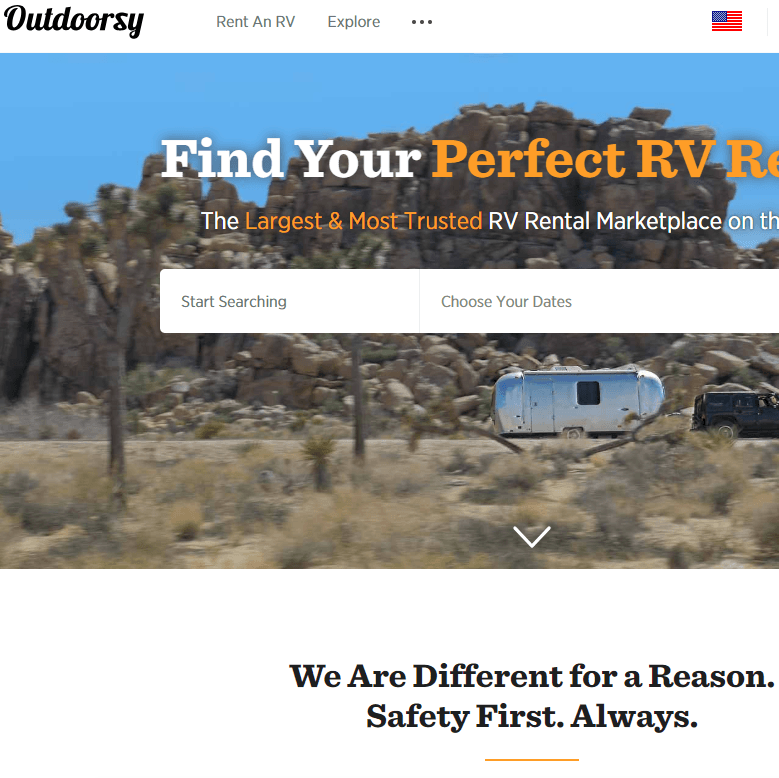This screenshot captures the landing page of a website named "Outdoorsy." The layout includes the platform's branding and purpose: an RV rental service. At the top, the word "Outdoorsy" is prominently displayed beside an icon of three dots and an American flag. The page encourages visitors to "Rent an RV" and "Explore." A striking image of a desert landscape under bright blue skies serves as the background, featuring rock formations, a trailer hooked up to a truck, and a few scattered trees and cacti, epitomizing a dry, rugged terrain.

The text on the page aims to guide visitors through the RV rental process. Below the header, a bold statement reads: "Find your perfect RV," with "Find your" in white and "Perfect RV" in a vibrant orange-yellow. The call-to-action continues with, "The largest and most trusted RV rental marketplace," accompanied by two interactive boxes inviting users to "Start Searching" and "Choose Your Dates." Beneath the "Choose Your Dates" box is a white arrow, likely indicating further action or navigation.

Additionally, a highlighted safety assurance is provided, reading "Safety First Always" underlined in yellow. The bold tagline "We're different for a reason" is written in black on the landscape image, emphasizing the company's unique value proposition alongside the detailed look and feel of the enchanting desert backdrop, merging practicality with the promise of adventure.